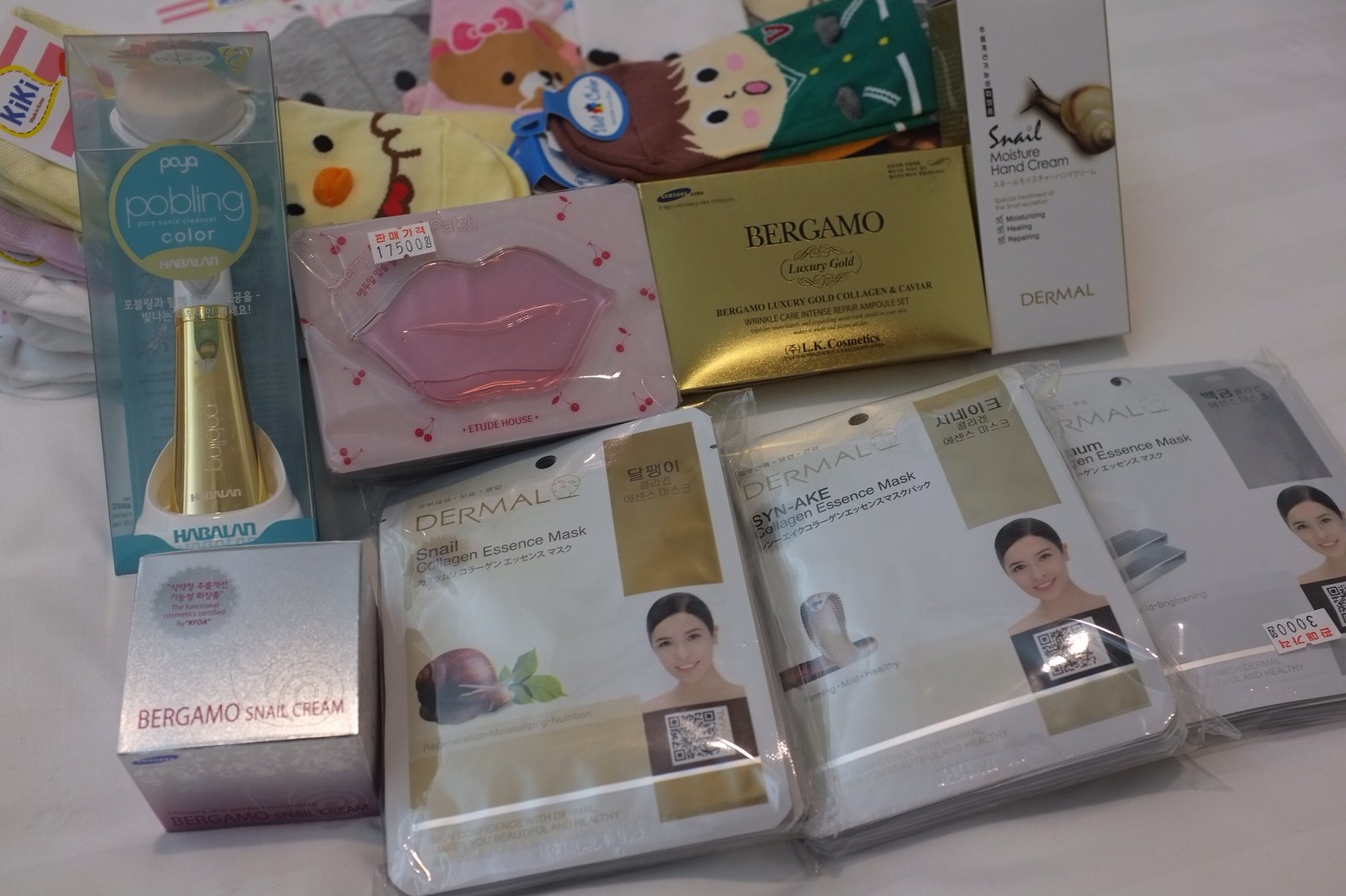The photograph captures an eclectic assortment of items arranged on a white sheet. In the background, an array of character socks can be seen, adding a whimsical touch to the scene. There is a pair of socks featuring a cheerful yellow duck with an orange beak, black eyes, and a red bow tie. Another pair displays a cartoonish human-like figure with brown hair, a green sweater adorned with gold buttons, and a comically open mouth shaped like an "O." Additionally, light pink socks showcase a bear's face, complete with a pink bow on its head.

Among the various cosmetic items prominently positioned, there is a gold tube and a pink lip product encased in a cherry-themed package. Another notable item is a gold package labeled "Snail Moisture Hand Cream" in black font, accompanied by an image of a snail. Adjacent to it, a silver box inscribed with "BERGAMO Snail Cream" in red font is also present. Further contributing to the skincare theme, several snail essence masks are included, featuring a smiling model with her hair pulled back. Some of these packages still bear price tags, emphasizing the new and ready-to-use nature of the products.